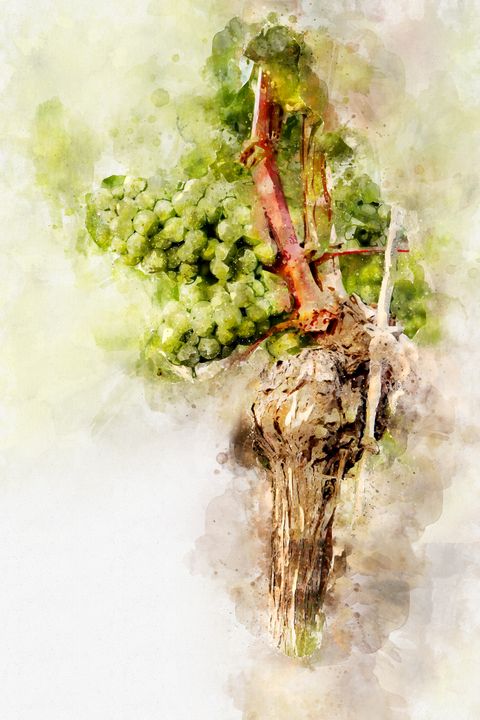This image appears to be a watercolor painting portraying a plant that shares features with both root vegetables and fruit-bearing vines. The painting has a predominantly white background, with shades of green, brown, and hints of red adding depth and detail. At the center, there are clusters of round, green objects resembling grapes, connected by brown stems and sticks, suggesting vine-like structures. Below, there is a brown and white area indicating a root structure with fine, white hairy fibers and remnants of brown soil clinging to it. This root structure transitions into a thick, orange-brown stem. The painted elements extend upward towards the top of the image, with gray hues partially surrounding the roots and grapes. The entire image appears to be presented behind a partially opaque or fogged sheet, possibly resembling cellophane or parchment, giving it a slightly obscured and pressed appearance, as if part of a display.